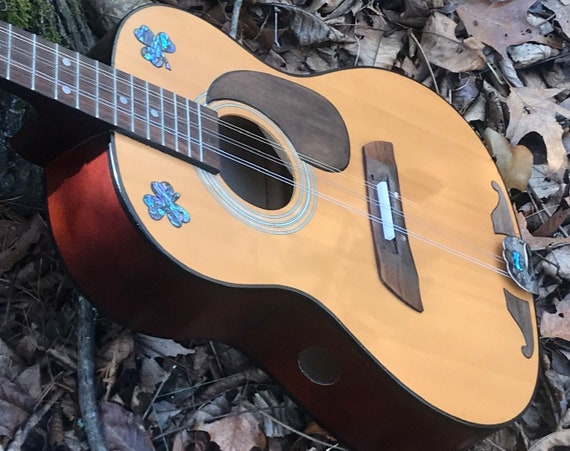The photograph is a digital close-up taken outdoors during the daytime. It features an acoustic guitar resting on a ground blanketed with dried leaves and twigs. The guitar has a natural wood-colored body with a darker brown fretboard and bridge. The neck of the guitar extends to the upper left-hand corner of the frame, partially overlapping the base of a tree trunk that is covered in green moss and appears dark gray. The guitar's face is adorned with two reflective clover stickers in metallic blue and purple, one on the upper left and one on the upper right side near the neck. The border of the guitar is a rich redwood hue, and there's a typical sound hole in the very center of its face as well as an unexplained hole on the lower half of its side. The image includes a palette of natural earth tones: shades of brown from the guitar and the surrounding leaves, with accents of green from the moss and the multicolored clovers. There is no text visible in the image, suggesting a serene, undisturbed setting in a wooded area.